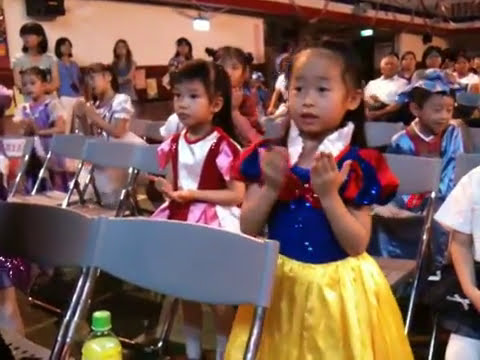The image depicts an indoor auditorium setting filled with many children, predominantly of Asian descent, and a few adults. The children's chairs are arranged in rows, featuring silver arms and legs with gray backrests. At the center foreground, a little girl dressed as Snow White stands out with her yellow skirt, blue bodice adorned with a red bow, puffy sleeves, and a white stand-up collar. She has dark eyes, dark hair, and is either clapping or about to clap. Beside her, another young girl sits wearing a pink and white princess gown, gazing upwards. Other children, some clapping and others looking around, occupy the rows behind them. A little boy in a blue hat sits among them, not looking at the performance like the others. Adults, likely parents or teachers, are positioned around the auditorium's edges, overseeing the scene. The photograph is in landscape orientation and captures a moment of vivid and realistic detail.